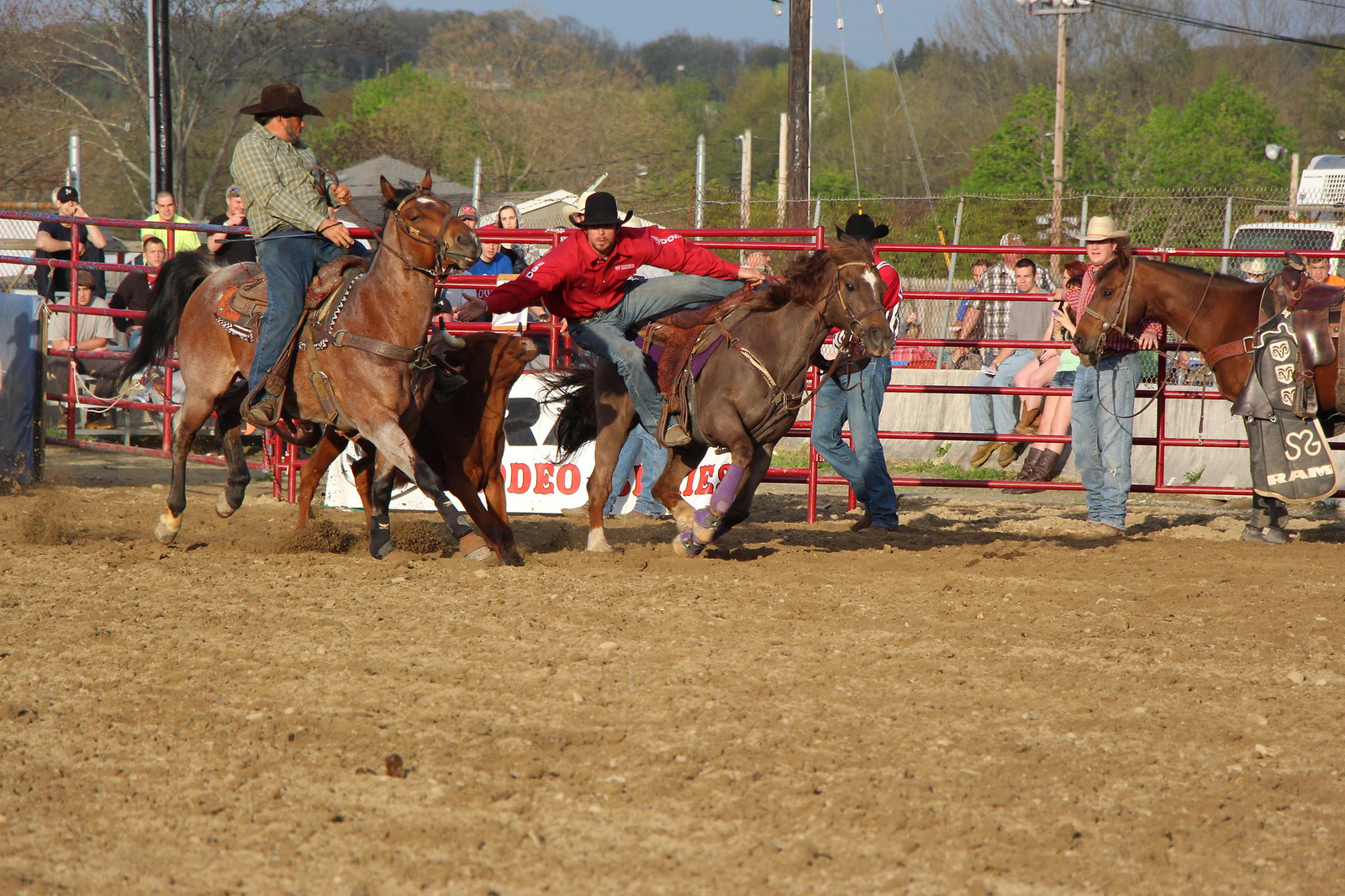This color photograph captures a dynamic moment at a calf roping competition held outdoors. At the center of the image, two men on horses flanking a calf are deeply engrossed in the action. The man on the left, clad in dark blue jeans and a green and white checkered shirt, guides his horse towards the calf. On the right, a second rider in a red sweater and dark blue jeans appears precariously positioned, almost falling off his horse as he reaches out. Another man in a blue hat watches closely, his horse standing nearby but not involved in the activity. To the side, by the red metal fence composed of horizontal bars, stands another horse, held by a man in a red and white checkered shirt, also wearing blue jeans. This man, along with another cowboy in denim and a red shirt, is observing the competition. The photo's background reveals a set of spectators seated on bleachers or chairs, while the very rural backdrop features a thicket of trees and a few visible power lines under a clear blue sky. The foreground of the image showcases the dusty, brown dirt of the rodeo arena, emphasizing the intensity and movement within the scene.